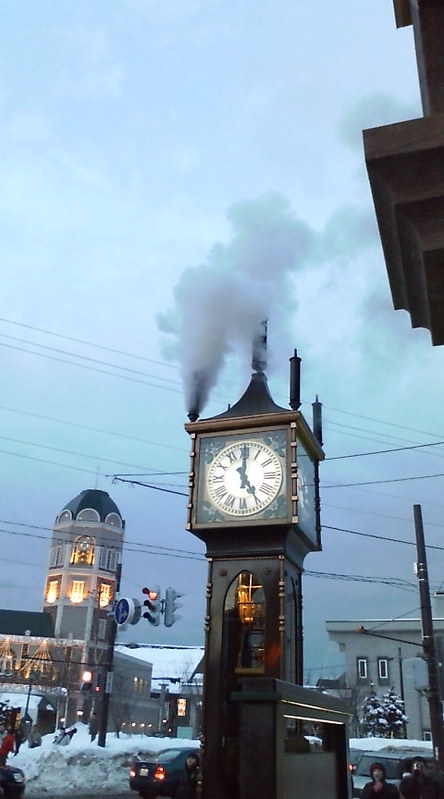In this outdoor image, a focal clock tower stands prominently in the center, contrasting against a sky painted with shades of gray, blue, and purple. The clock tower, resembling a Victorian-style grandfather clock, is quite tall, estimated to be around 15 feet high, and has a rectangular base transitioning into a cube at the top. The tower is primarily dark brown and gray, with glass windows encasing its sides and front. The striking white clock face displays Roman numerals and ornate black hands, framed by a glass cover.

Atop the tower, there are four chimney-like stacks, designed to emit thick gray smoke, adding a steampunk element to the scene. One of these stacks actively releases smoke, likened to smog. The clock is also a steam exhaust mechanism, making it a unique feature in the landscape.

The surroundings hint at a European city, possibly Eastern Europe or Britain, as suggested by the style of streetlights, signs, and architecture. Snow banks line the sidewalk where a few pedestrians are visible, hinting at recent heavy snowfall. Cars and power lines are also seen in the background. 

An interesting building with a dark dome is observed behind the clock tower, and there’s also a white flat-roofed building on the bottom right side of the image. The atmosphere of the scene is cold and wintry, with the clock showing five o'clock.